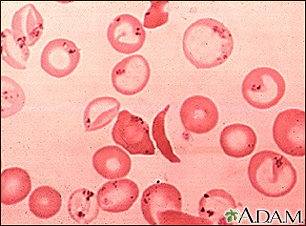The image appears to be a highly detailed, monochromatic depiction of cells or microscopic life forms, rendered in varying shades of red, pink, and cream. These forms float against a light pink or gradient background, some appearing solid while others have open or dotted interiors. They generally take on round or oval shapes, though their edges are rough and some are deformed, resembling blood cells or other microscopic elements. Notably, there is a watermark in the bottom right corner featuring the text "ADAM" next to a logo that resembles a leaf or a palm tree. The overall texture of the image seems grainy, hinting at either a photographic proof, a digital scan, or an artistic representation of these biological forms.